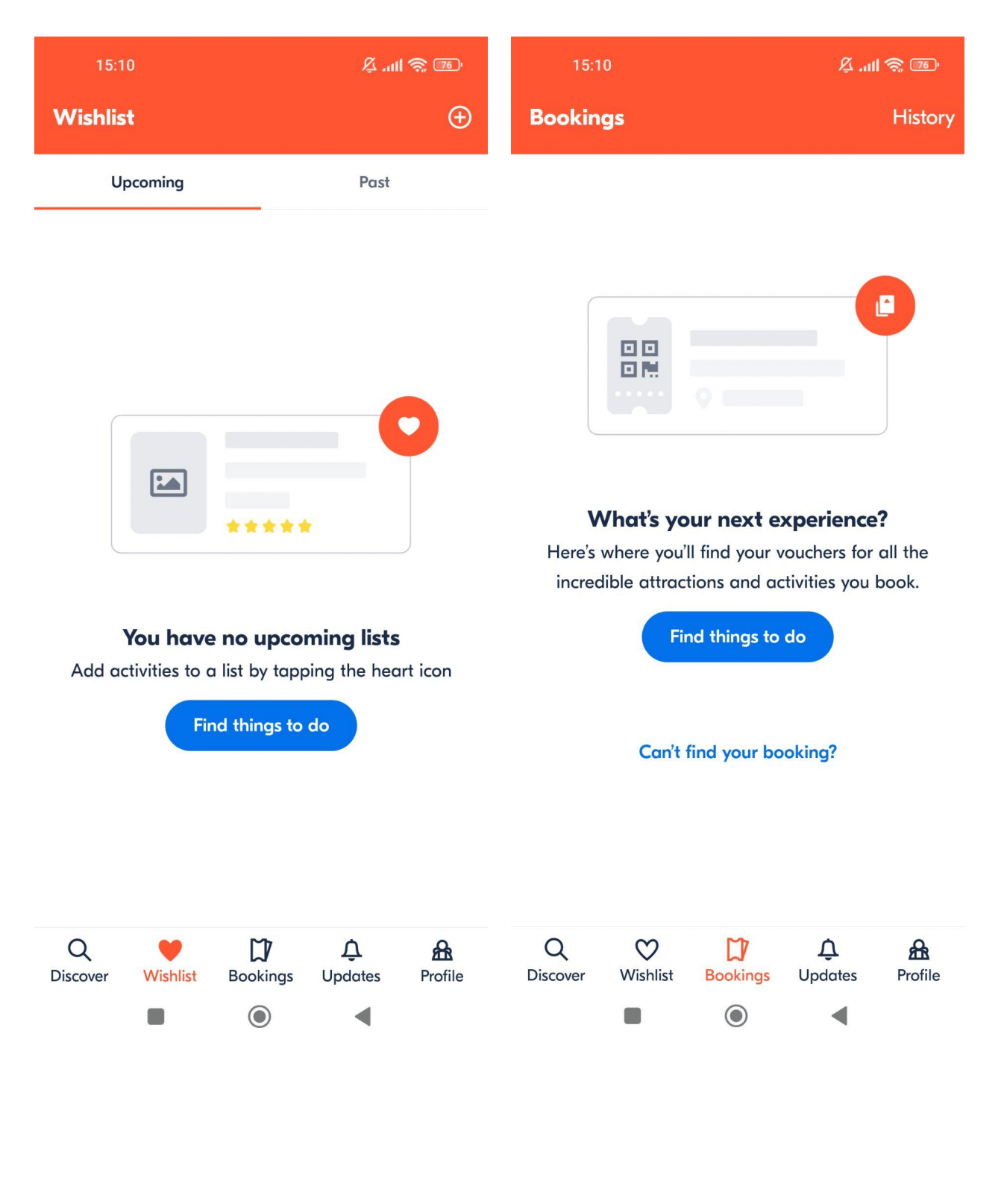The image is a side-by-side screenshot comparison from a mobile application. Both screenshots show the top section of a phone screen, with the battery indicator approximately three-fourths full and the time displayed as 3:10 PM.

In the left screenshot, the user is on a "Wishlist" screen specifically in the "Upcoming" tab. The interface shows a message stating, "You have no upcoming lists," and instructs users to "add activities to a list by tapping the heart icon." Below this message, there is a prominent blue button labeled "Find things to do." Additional tabs labeled "Past," "Bookings," and "History" are visible in the top navigation bar.

The right screenshot displays the "Bookings" tab. The screen is titled "What's your next experience?" with a subheading instructing users that they can find vouchers for all their booked attractions and activities here. A blue button labeled "Find things to do" is prominently featured. Below this button, there is text that reads "Can't find your booking?" followed by navigational options for "Discover," "Wishlist," "Bookings," "Updates," and "Profile," with "Bookings" highlighted to indicate the current active tab.